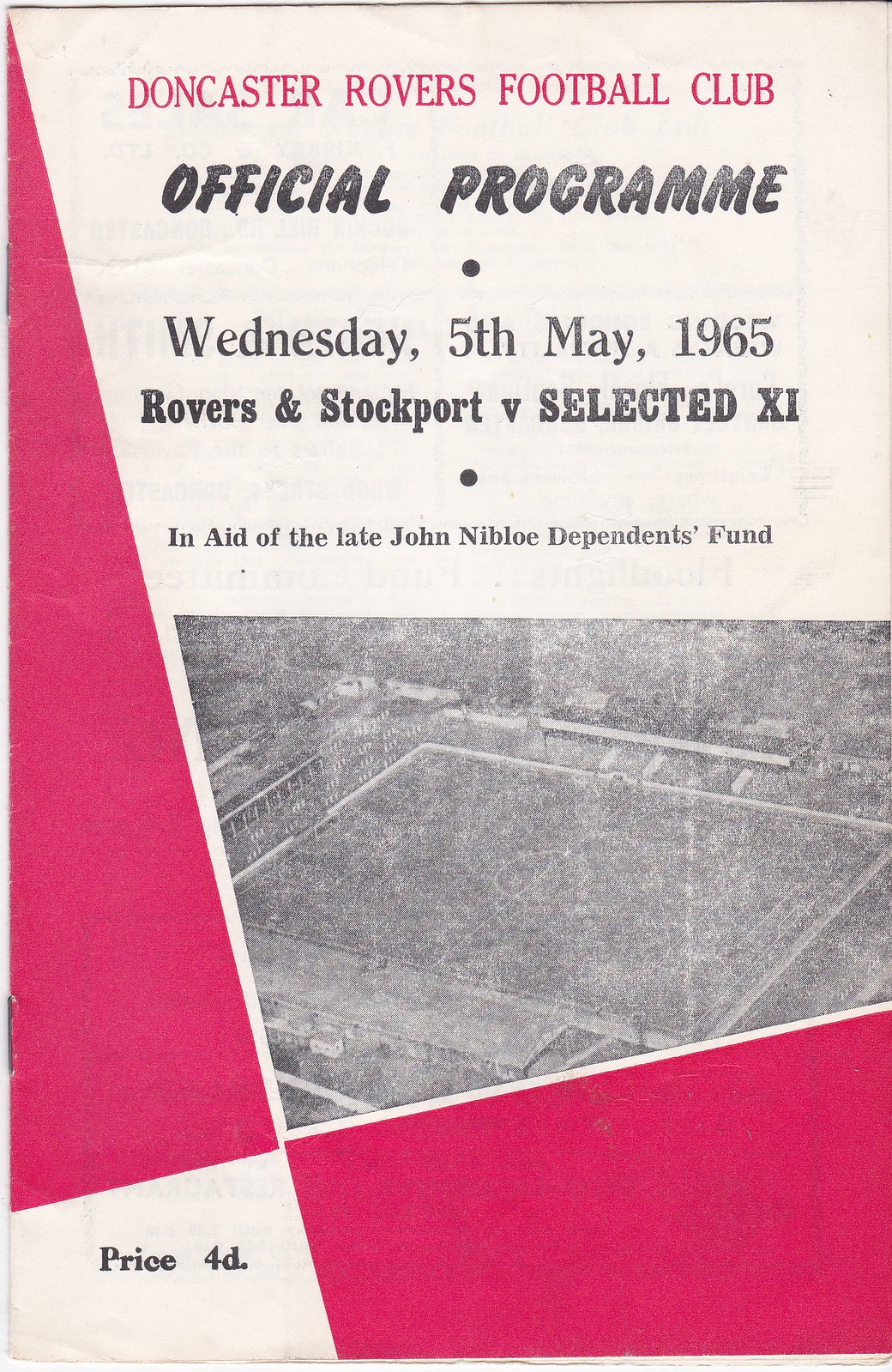This image depicts a historical sports program for a soccer match featuring the Doncaster Rovers Football Club. The program, dated Wednesday, the 5th of May, 1965, prominently displays the club's name in red at the top. Below this, the text "Official Program" is printed in black. The event is noted as a match between "Rovers and Stockport versus Selected XI" and is in aid of the late John Niblo Dependents Fund. The design includes a distinctive red triangular pattern running along the left side and the bottom right corner, with the text "Price 4D" between the two red blocks. A faded black and white photograph, presumably of the stadium, is centrally featured on the cover, contributing to the vintage appearance of the program.